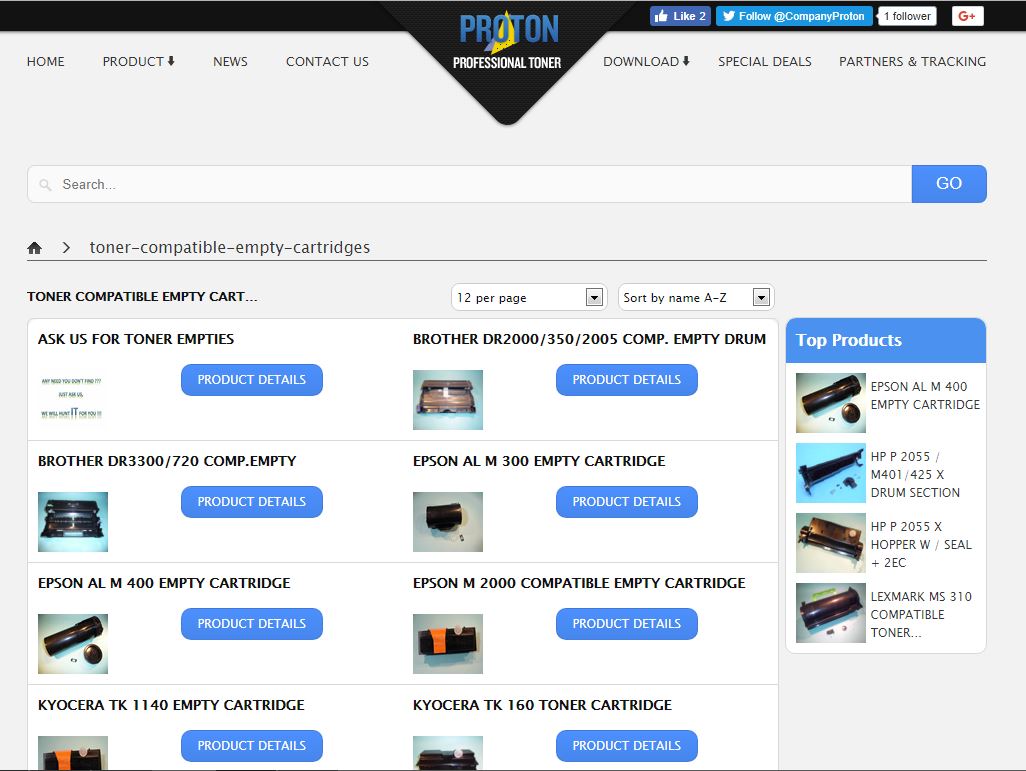**Detailed Image Caption for Website Category:**

The image showcases a website layout under the "Websites" category. At the top of the page, there is a prominent black bar featuring a centered, downward-pointing triangle. Inside this triangle, the text "Proton Professional Toner" is displayed, accompanied by two likes and one follower.

Beneath the black bar is a grey navigation area listing several menu options: "Home," "Product," "News," "Contact Us," "Downloads," "Special Deals," and "Partners in Tracking." Just below this menu is a search bar, equipped with a magnifying glass icon and a blue "Go" button.

Further down the page, an icon resembling a small house appears next to the text "Toner Compatible Empty Cartridges." Additional text reads "Toner Compatible Empty Cart," followed by options to display twelve items per page and to sort products by name from A to Z. There is also a prompt: "Ask Us for Toner Empties" and a link to "Product Details," though no image accompanies it.

Subsequently, a list of toner-related products is displayed:
- Brother DR3300 Compatible Empty Cartridge (Product Details)
- Epson AL400 Empty Cartridge
- Casera TK1140 Empty Cartridge
- Brother DR2000 Empty Drum
- Epson AL Empty Cartridge
- Epson 2000 Empty Cartridge